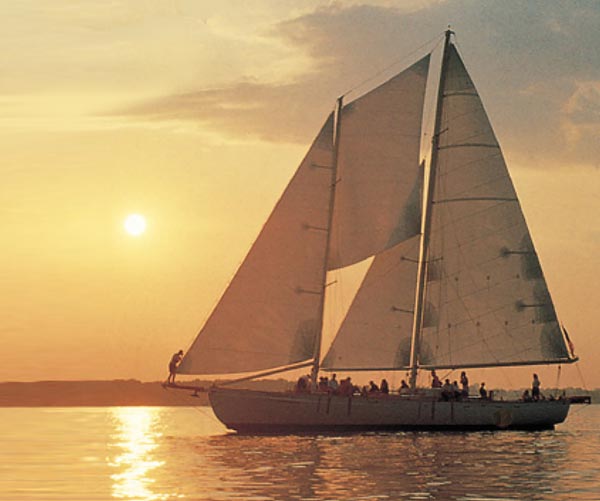The image captures a beautiful, medium-sized sailboat on a calm ocean during what appears to be sunset on a sunny day. The entire scene is bathed in shades of tannish gold, with hints of orange, red, and blue from the setting sun and scattered clouds. The sailboat has three tall masts with sails – two triangular and one rectangular. There are approximately 20 people depicted on the boat, all shown in silhouette or shades of brown, lacking detailed features. A man is standing at the stern of the boat, seemingly repairing one of the sails. In the background, rolling hills or a shoreline with trees and foliage are visible on the horizon. The water is very still, reflecting the bright white orb of the sun in the sky. The overall ambiance is serene and picturesque, showcasing the sailboat elegantly gliding through the tranquil waters.